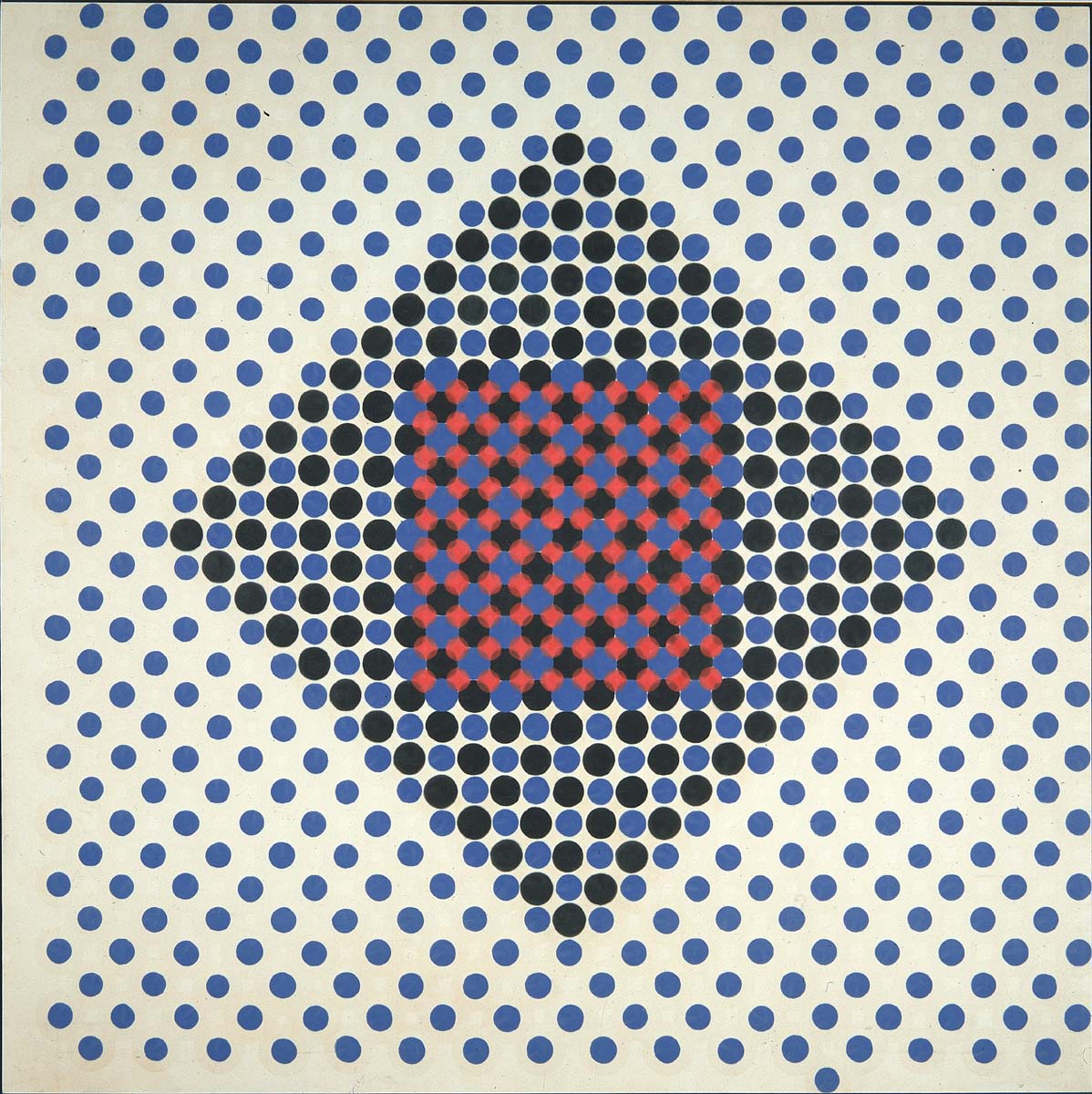The image is a detailed drawing focusing on intricate designs composed of various dots and squares. The background of the image is either white or cream, setting a soft contrast to the vibrant elements on it. Predominantly, dark blue dots are evenly spaced and arranged in diagonal, vertical, and horizontal lines across the image. The centerpiece of the design features a diamond shape formed by black and blue dots, with the black dots being notably larger. At the heart of this diamond is a square, distinguished by its densely packed black and blue dots, complemented by an X pattern made of red dots. The overall arrangement creates an intriguing optical illusion, blending different shapes and colors into a captivating visual display.